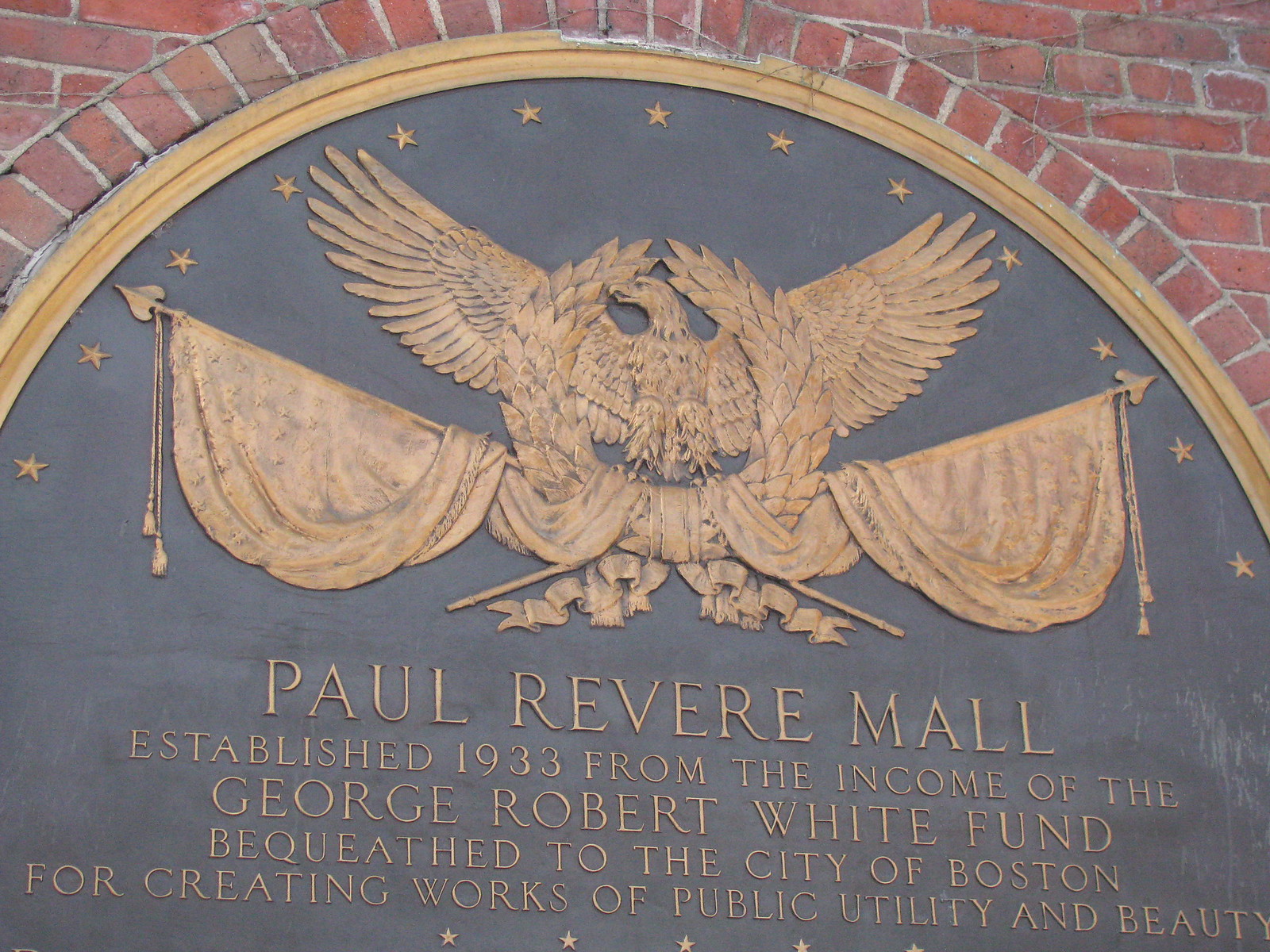The image depicts a historical plaque set into a circular section of an aged brick wall, suggesting it is part of the entrance to the Paul Revere Mall. The plaque features a gray-blue background with a gold border and contains several intricate elements in gold. Centrally, it showcases an eagle with wings outstretched, surrounded by a wreath and accompanied by draped cloth and banners. Above the eagle, there are gold stars, adding to the commemorative design, while beneath it runs a row of additional stars. The text on the plaque reads, "Paul Revere Mall, established 1933 from the income of the George Robert White Fund, bequeathed to the city of Boston for creating works of public utility and beauty." The surrounding brick wall arches above the plaque, enhancing its prominence, and displays signs of age, such as spiderwebs and twigs.